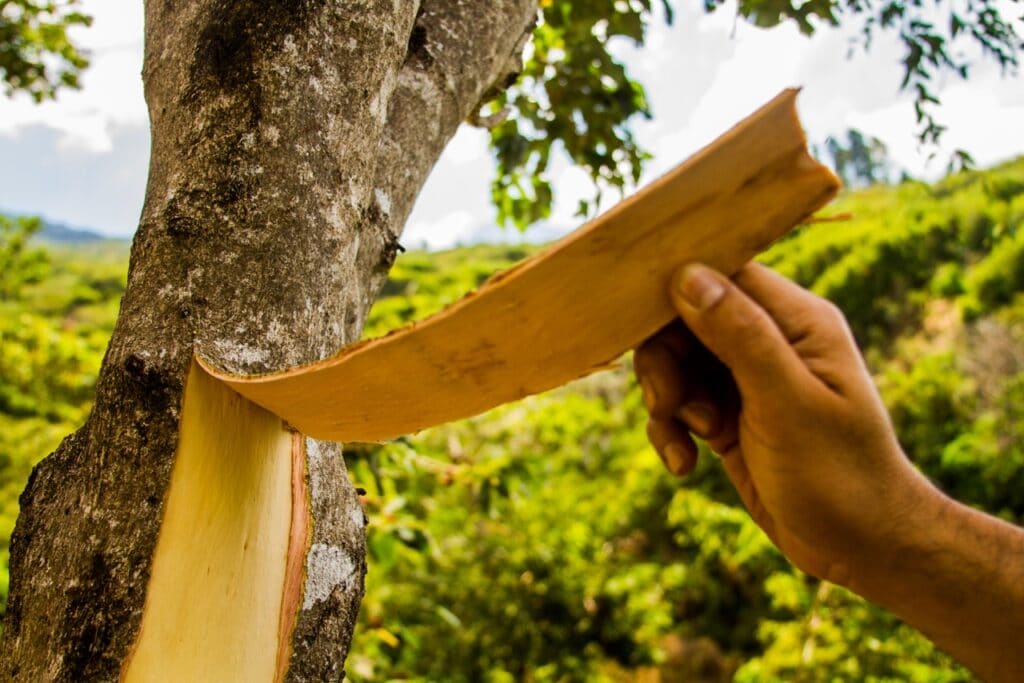A detailed photograph highlights an individual carefully peeling a piece of bark from a relatively young tree. The exposed inner wood reveals a yellowish hue, contrasting sharply with the textured, aged bark adorned with patches of moss. In the background, a sunlit meadow gently rolls over a hill, though it appears soft and out of focus. The sky above carries dark, looming clouds, suggesting an impending change in weather, yet the current scene is kissed by sunlight, casting warm reflections on the tree and the person's hand. The out-of-focus leaves form circular, bokeh-like patterns in the backdrop, adding a dreamy quality to the image. The overall warm tones and the lush greenery of the meadow create a tranquil and inviting atmosphere.